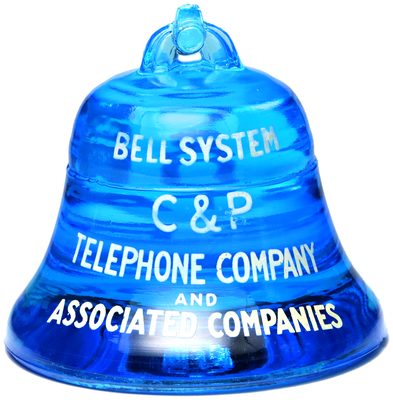This image features a meticulously polished, translucent blue bell that appears to be made of glass or crystal. The bell showcases a gradient of blue shades, transitioning from a darker, ocean blue at the base to a lighter, sky blue towards the top. The bell has horizontal striations encircling it and is topped with a curved handle, complete with a small knob or button at its peak. Across the bell, white text reads: "Bell System" at the top, followed by "C&P Telephone Company" below, and ending with "Associated Companies" at the bottom, with each phrase descending in size. The overall appearance is reminiscent of an old-fashioned advertisement, yet the image contains no additional context or background, focusing solely on the elegant simplicity and smooth texture of the bell.